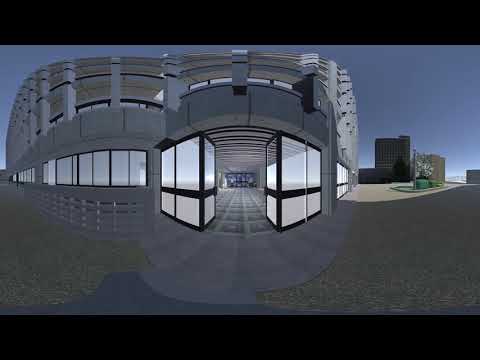The image showcases a detailed, computer-generated architectural scene, centered around a large, multi-story building with noticeable windows and an open entrance revealing part of the interior. The scene appears to be designed using 3D graphics, resembling a fisheye lens view that adds a warped, interactive quality to the image. The setting is outdoors in the middle of the day, enhanced by a luminous light source positioned out of frame to the right, causing light to fall on the concrete walkway in front of the building. The background features additional buildings and a clear blue sky without clouds. The colors in the image mainly comprise black, gray, blue, light blue, green, and brown, set against solid black borders at the top and bottom. No text or people are present within this detailed digital architectural visualization.